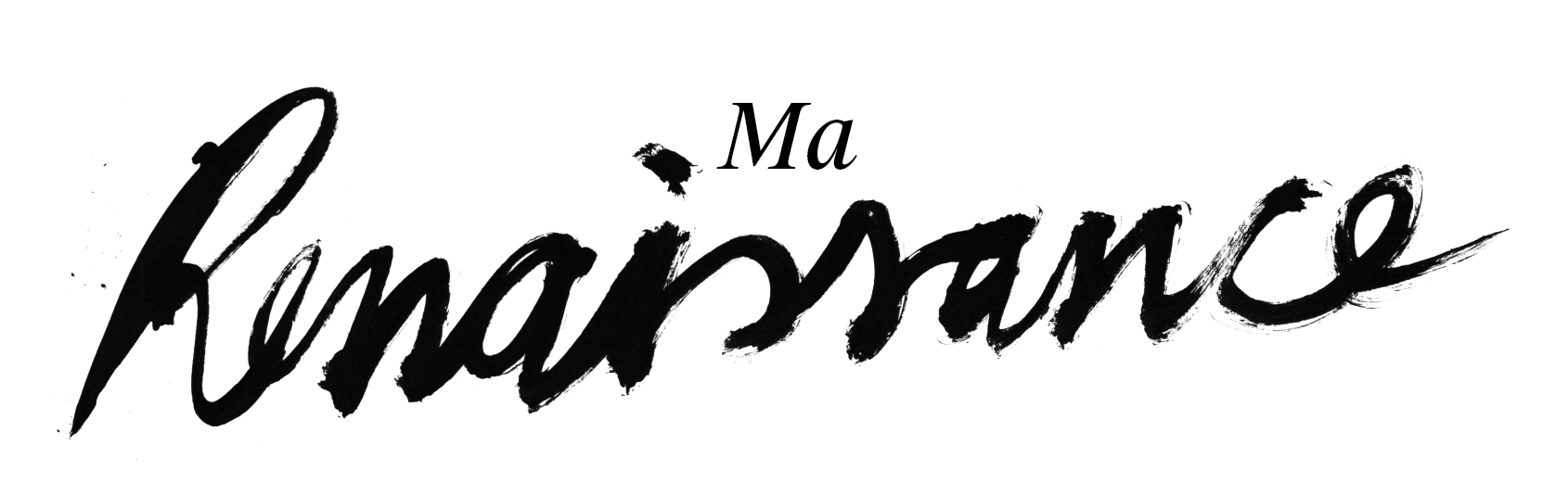The image features a completely white background with text in two distinct styles. At the top, the letters "MA" are typed in a light black or dark gray color, resembling a computer typewriter font. Directly beneath this, the word "Renaissance" is handwritten in black cursive paint, with a clearly defined dot above the "i". The cursive word starts lower and tilts upward, giving it a dynamic, ascending look. The second "e" in "Renaissance" is the only letter that appears solidly straight. The overall composition is simple, with just these two elements – "MA" in a clean, typed font and "Renaissance" beneath it, artistically painted in cursive – set against the pristine white background.